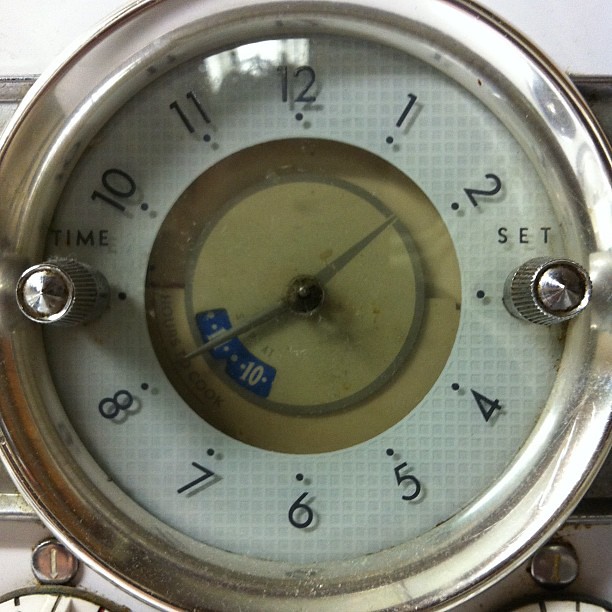This image is a detailed close-up of an old-fashioned clock, likely from a stove, with a dusty chrome finish. The face of the clock is primarily white, featuring large black numbers and two equal-sized silver hands indicating the hour and minute. The area around the hands has a pale yellowish tint. The top center of the face reads "hours to cook," suggesting a kitchen appliance origin. Two silver buttons are visible: the left button is labeled "time," and the right button is labeled "set." Both buttons flank the clock face symmetrically. Visible signs of use, such as grease and food marks, are present, particularly around the buttons and dials. The clock appears dirty, with grease spots and dents in the glass. In the bottom right corner, a partial view of a stove dial is seen, reinforcing the likely association with kitchen equipment. Overall, the clock exudes an antique vibe and seems to have been well-used in its setting.